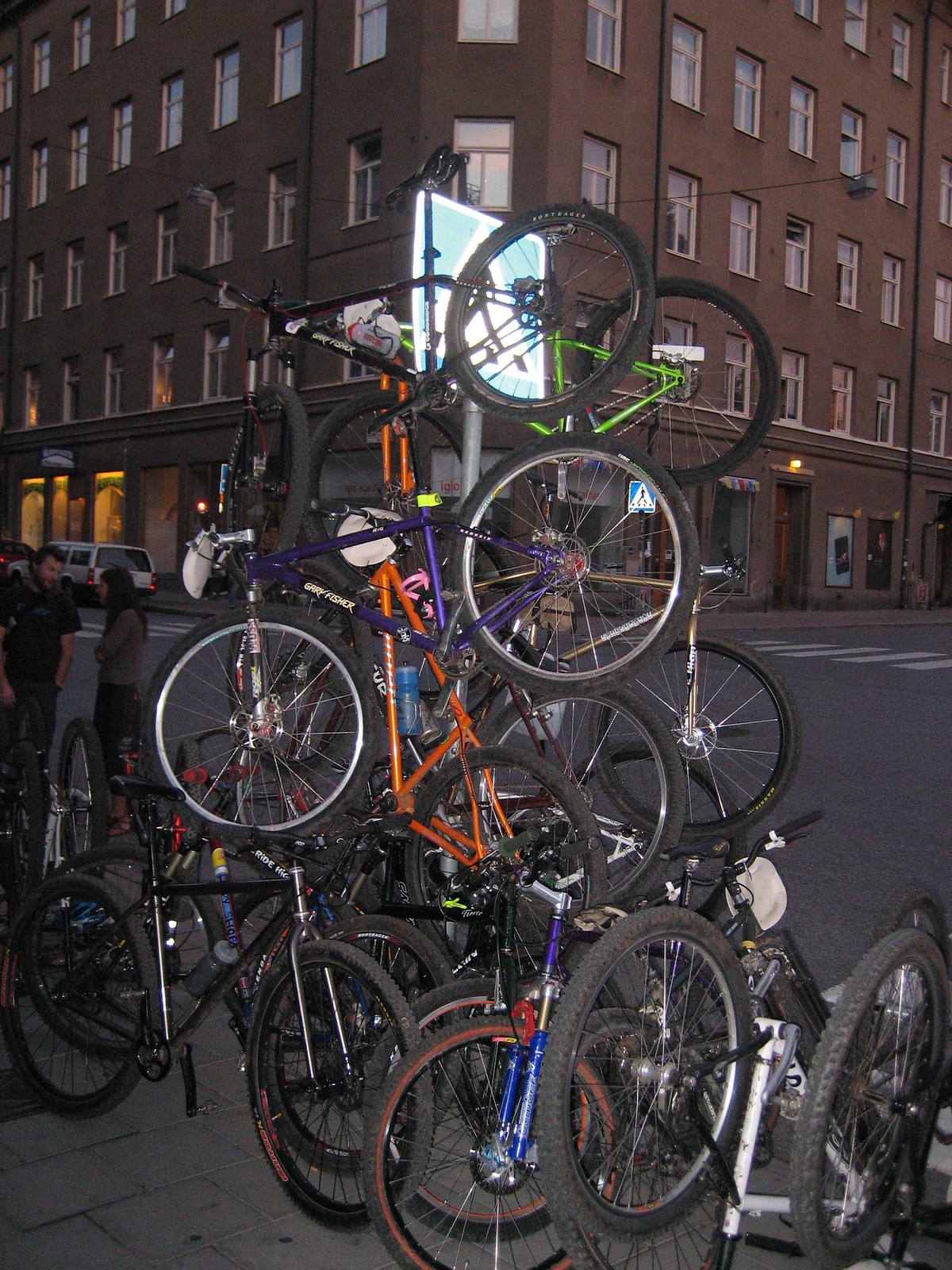In this photograph, a chaotic mountain of bicycles dominates the scene, showcasing at least four layers of bicycles stacked wildly on top of one another. The vivid array of bicycles includes orange, black, green, blue, and purple ones. At the base, several bicycles are parked normally on their stands or lying haphazardly on the sidewalk, but as you move upwards, they become more intertwined and disorganized, creating a striking visual centerpiece. The background features a large brown building that spans the entirety of the upper half of the image, likely an apartment complex or shopping center, with numerous windows, doors, and shop fronts. On the left side of the frame, a man in a short-sleeved black t-shirt and a woman in a gray sweater, distinguished by their dark hair, add a human element to the bustling urban scene. The photograph captures the vibrant and somewhat chaotic essence of city life through this intriguing pile of bicycles.